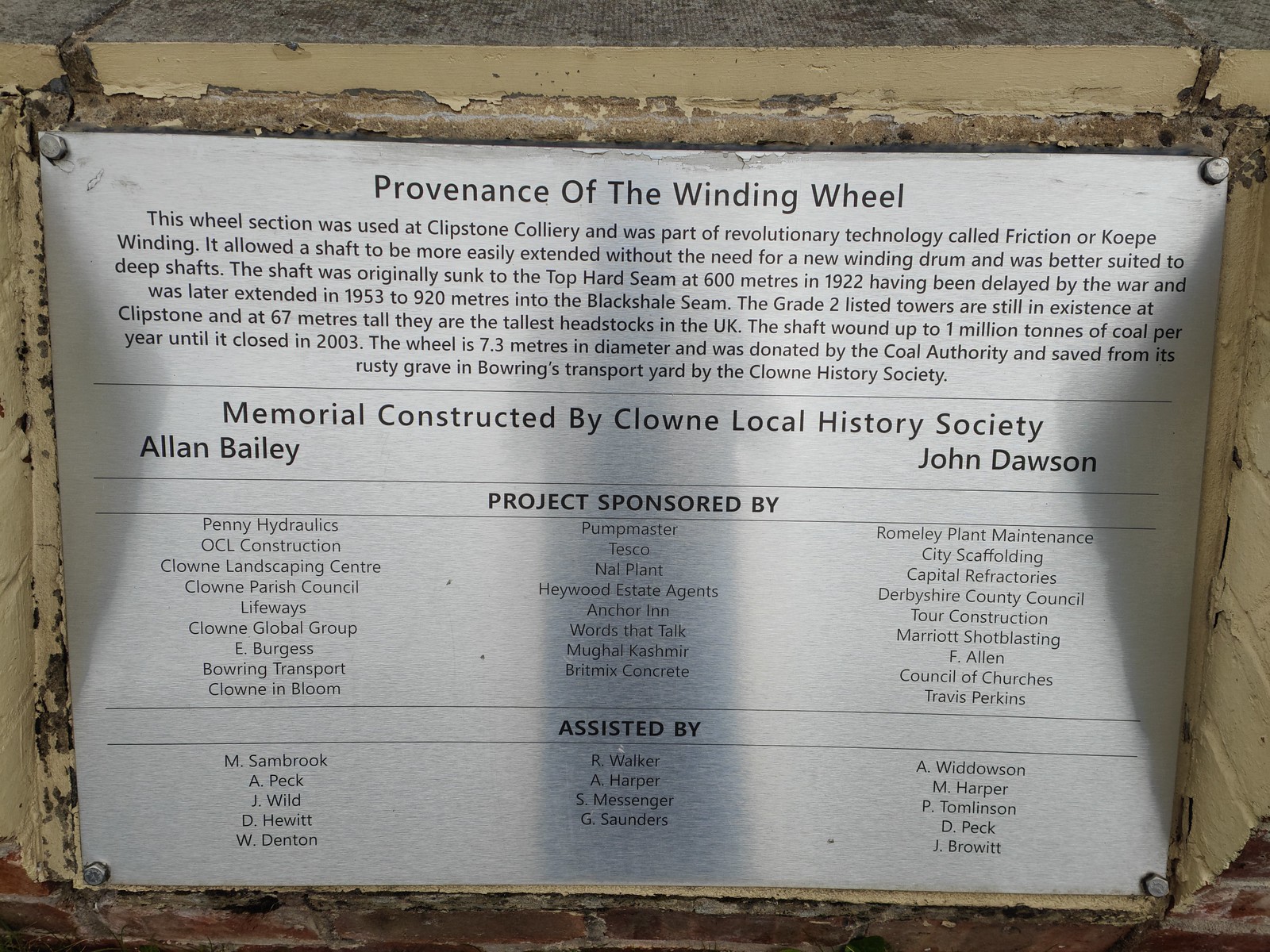The plaque, mounted on a deteriorating yellow-painted cement wall, commemorates the "Province of the Winding Wheel." The wall shows significant wear, with chipping paint revealing signs of aging. The plaque is bordered by wood and provides detailed historical context about the wheel section, originally used at Clipstone Colliery. This section was part of a revolutionary technology called friction or cope winding, which allowed shafts to be extended more conveniently without needing a new winding drum. Specifically, the shaft was first sunk to the Top Hard seam at 600 meters in 1922 but was delayed by the war. It was later extended in 1953 to 920 meters into the Black Shale seam. Notably, the Grade II listed towers at Clipstone, standing at 67 meters tall, are still intact and are the tallest headstocks in the UK. Impressively, the shaft wound up to 100 million tons of coal per year until its closure. The memorial was constructed by the Clown Local History Society, with contributions from Alan Bailey and John Dawson. The project was sponsored by three columns of various individuals and entities, including Penny Hydraulics, and additionally, four to five names per column are listed as having assisted with the project.